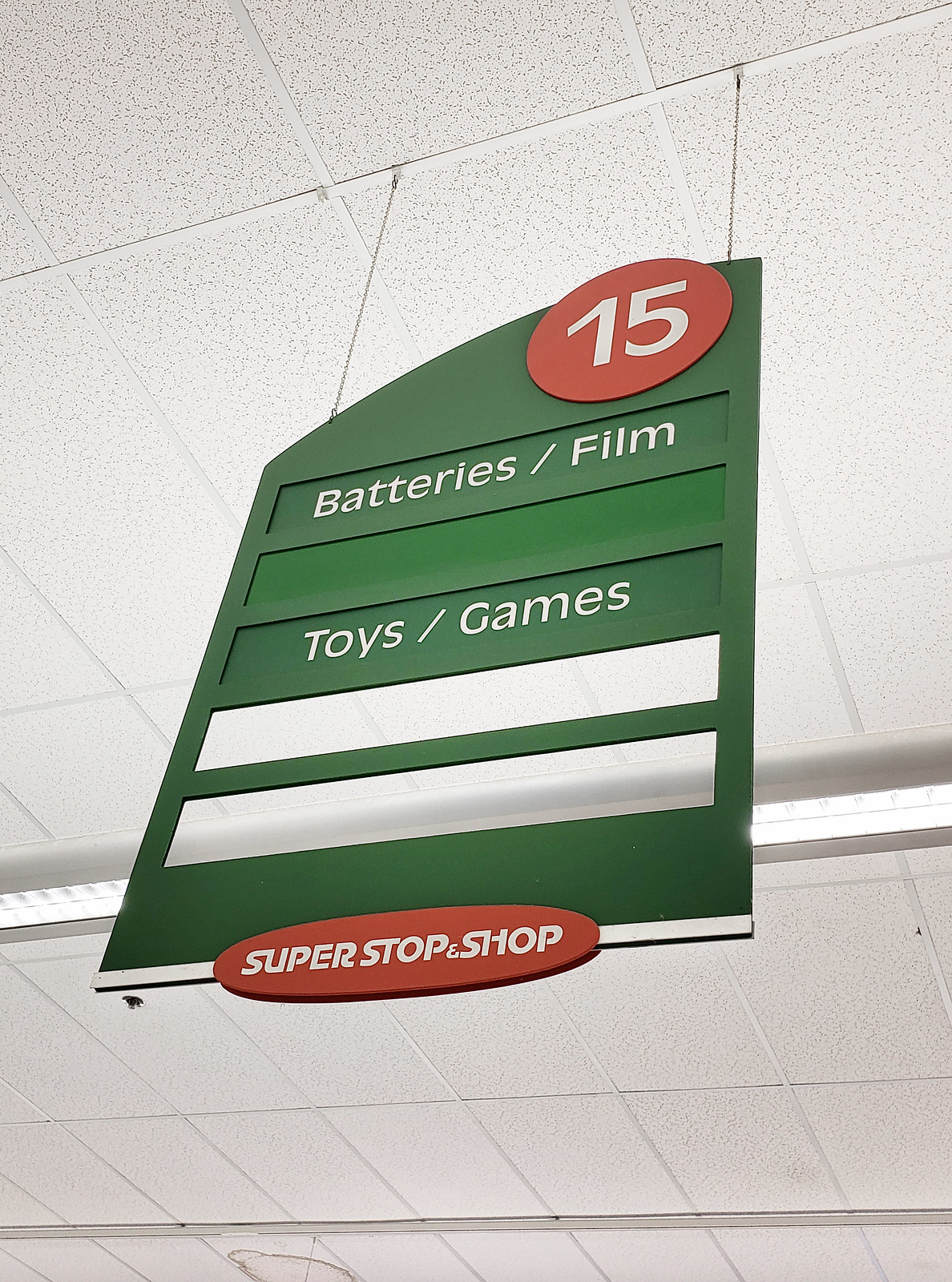A green aisle marker sign hanging from the ceiling at Super Stop-and-Shop. The sign is suspended by wires from a drop-down ceiling. Its top has a curved design, while the bottom and sides are flat. A prominent red circle at the top displays the number "15" in white, indicating the aisle number. The sign lists categories such as "Battery/Film" and "Toys and Games," with some space between the words. At the bottom of the sign, within an oval shape, the store's name, "Super Stop-and-Shop," is prominently displayed. This sign clearly marks aisle 15 and guides customers on what products they can find there, along with the store's branding.